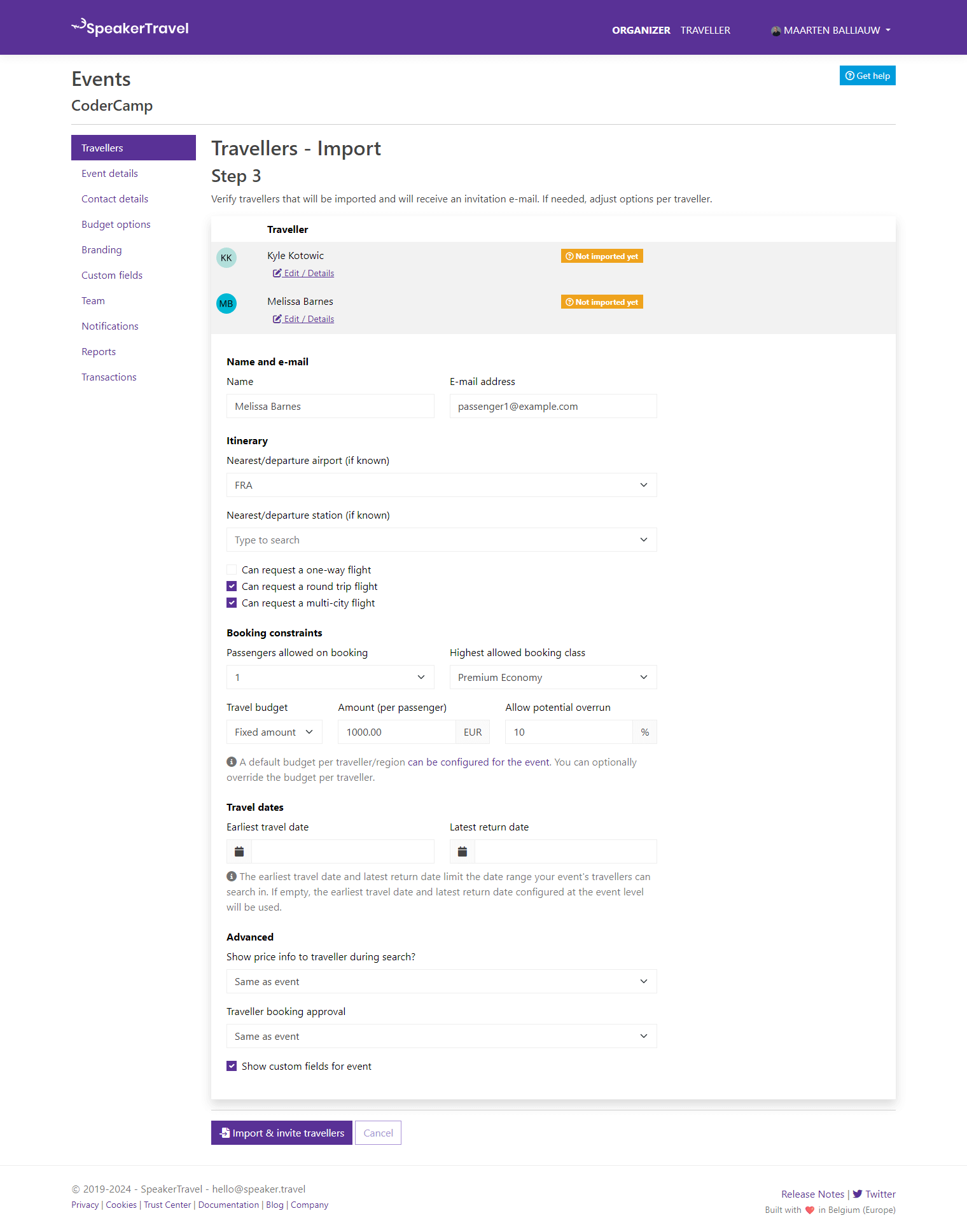Screenshot of a webpage featuring small, detailed text with various sections. At the top of the page, a blue rectangle with white text serves as a prominent heading. The page content is diverse, listing categories such as "Speaker," "Travel," and "Events," as well as specific elements like "Coder Camp," "Travelers," "Import," and "Step Three," each accompanied by checkboxes for user interaction. Near the bottom, a purple rectangle with white text, likely a button labeled "Send," is situated prominently. There is also a white rectangle nearby that appears to be another "Send" button. The very bottom of the page contains additional information, presumably including copyright details.